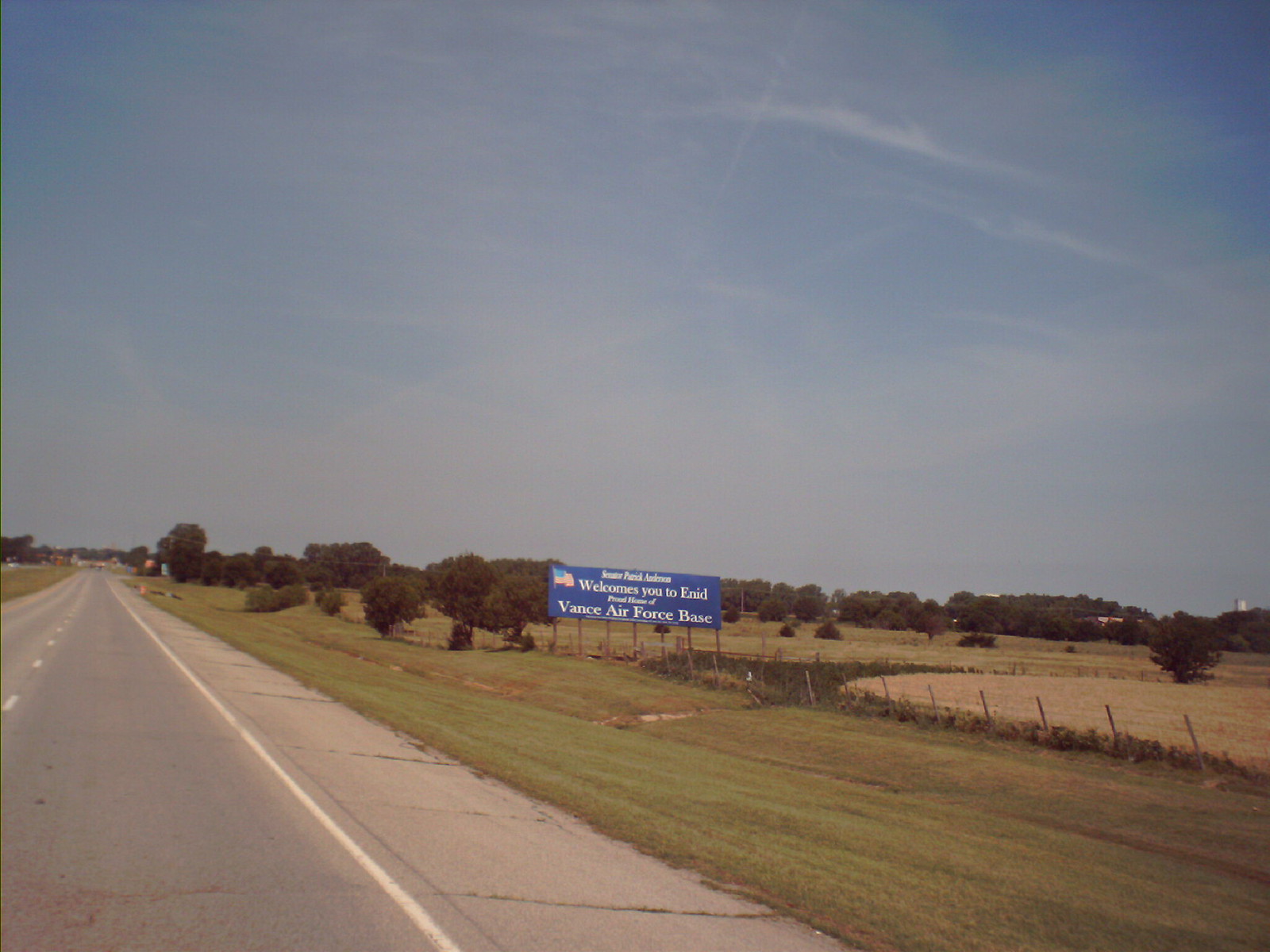This slightly grainy photograph taken from a moving car captures a sunny day along a concrete highway. The road, positioned about two inches from the left edge of the image, extends straight ahead and tapers into the distance. White dashed lines mark the road's center, while a solid white line runs along the right side next to a concrete barrier. Beyond the barrier lies a grassy area, interspersed with patches of brown dirt and a barely visible wooden fence with wire.

Central to the image is a prominent blue billboard adorned with white lettering and an American flag in the top corner. The sign reads, "Welcomes you to Enid" at the top, with "Vance Air Force Base" at the bottom, though some of the intermediate text remains illegible. The background features dense, bushy trees and dark green grass, seamlessly blending into a distant tree line adjacent to a railroad. The blue sky above is dotted with wispy clouds, adding to the idyllic outdoor setting.